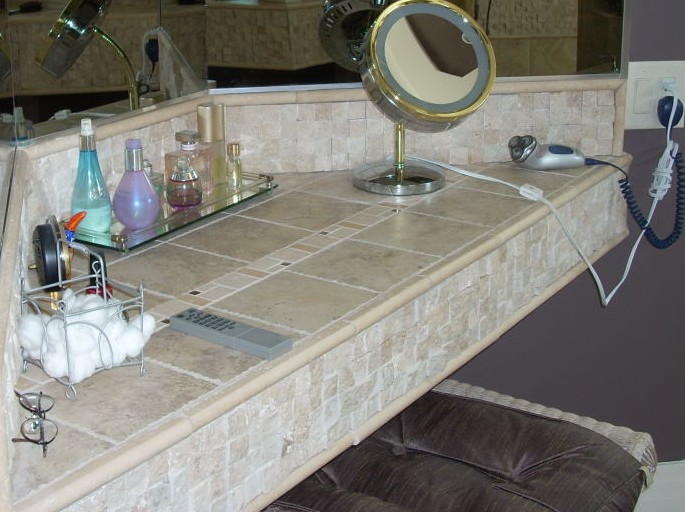This photograph, taken from an overhead perspective, captures an elegantly arranged bathroom vanity set in an alcove area, flanked by two graduated sides that meet centrally. The vanity's surface and front face are adorned with ivory square tiles, complemented by a matching square mosaic tile backsplash. A mirror spans the wall behind the vanity, amplifying the visual depth of the scene.

On the left-hand side of the vanity, a pair of wire-rimmed glasses sit folded flat beside a white wire basket filled with soft cotton puffs. Adjacent to the basket, the side of a wind-up style alarm clock peeks into view. The center of the vanity is adorned with a glass mirrored tray displaying an eclectic assortment of perfume bottles. Among them, a striking turquoise blue bottle with a white top, a delicate lilac purple bottle, and several clear glass bottles with gold or clear stoppers contribute to the charming array.

The right-hand side of the vanity features a sophisticated light-up makeup mirror, distinguished by its silver metallic base, gold-colored shaft, and brass-lined rounded face. Nestled beside it is a sleek, three-head electric shaver with a silver base. The functional elements are linked by a white plug from the mirror and a coiled black cord from the shaver.

In front of the vanity, a rustic-style bench with a plush brown velvet cushion, tufted for added texture and comfort, completes the refined and meticulously organized space.